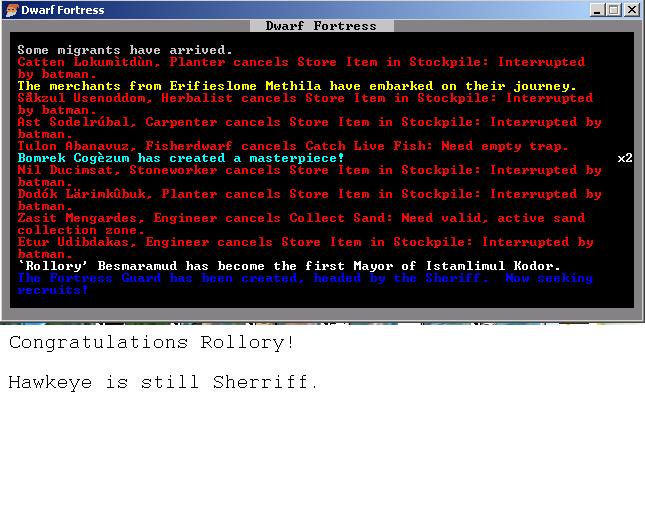The image displays a pop-up notification from the video game Dwarf Fortress on a computer screen. The background is black, providing a stark contrast to the colorful text. 

The main text in the notification includes:
- "Migrants of the Thrive: Gatton Lactoderm" 
- "Something Interrupted by Batman"
- "Merchants from Ihrlstam: Metcha have embarked on a journey"

In striking red text, there's a message about an interruption.

In blue text, it proudly states, "Bomb Rep Pogosam has created a masterpiece."

The red text continues with, "Valery Besmar has become the first mayor of Istanbul, Kodor."

At the bottom of the notification, it congratulates Valery with the message, "Congratulations, Valery. Hawkeye is still Sheriff."

The entire scene is captured on a black background, emphasizing the colorful notifications and creating a visually engaging narrative of events in the game.